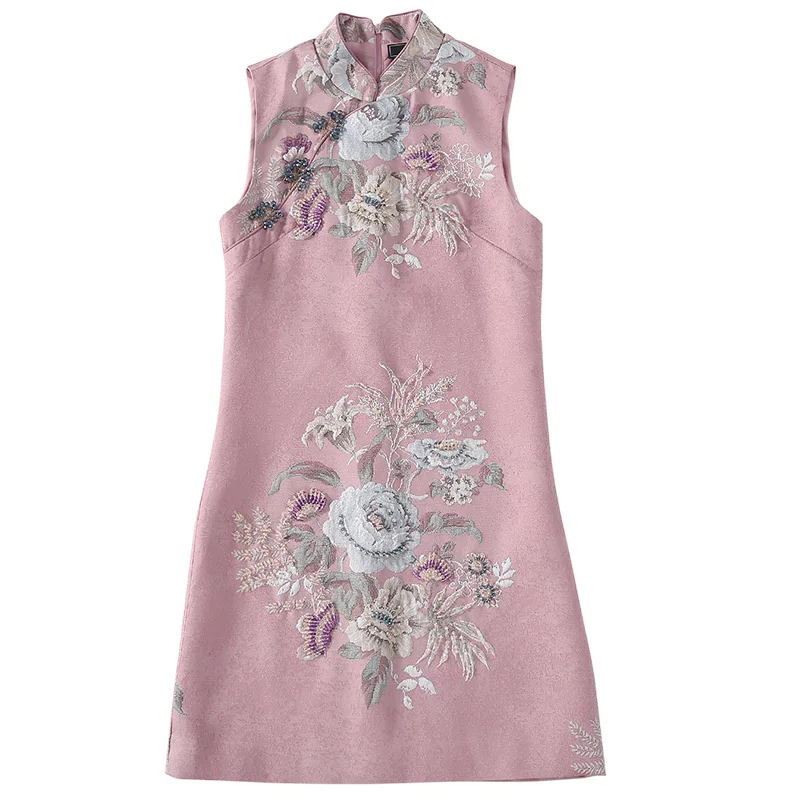This image showcases a high-quality, professionally photographed pink silk dress set against a crisp white background. The vertically oriented picture captures every intricate detail of the sleeveless, knee-length dress, which features a stand-up collar evocative of Asian design. The dress sports a fitted silhouette with subtle darts at the bustline, adding to its tailored look. Both the chest and stomach areas are adorned with an exquisite floral embroidery that includes a tapestry of red, pink, and white flowers alongside green leaves, enriched by gray and tan beading. This same intricate pattern is echoed around the middle section of the skirt, adding a harmonious touch of elegance and cohesion to the garment.